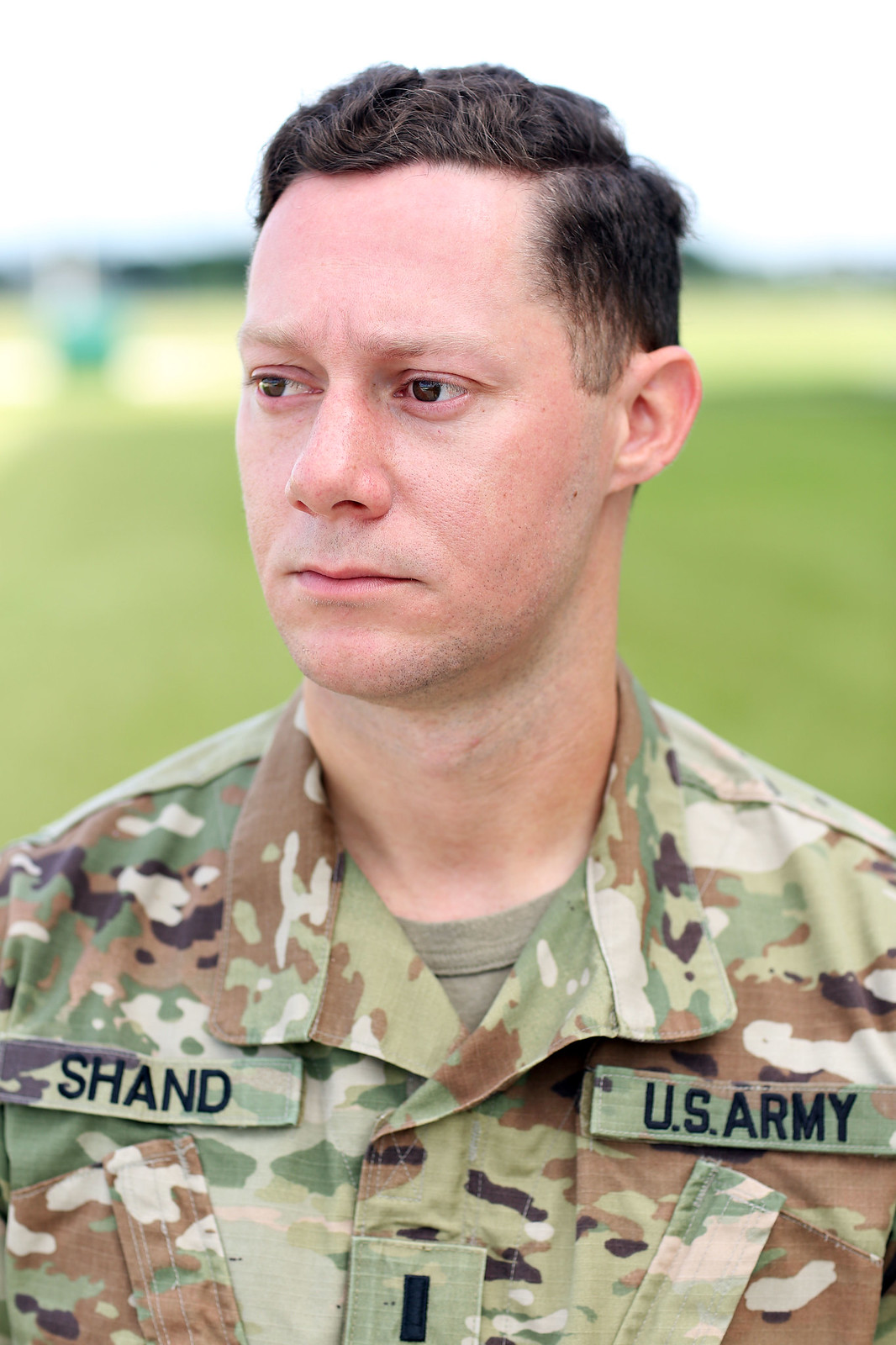This vertically-aligned color photograph captures a close-up of a somber-faced U.S. Army soldier named Shand. The soldier, centrally positioned in the image, has short brown hair, dark brown eyes, and a clean-shaven face. He is dressed in a camouflage uniform consisting of green, brown, and black colors, with a brown T-shirt underneath. The uniform prominently features two patches on the chest area: "SHAND" in black capital letters on the left pocket, and "U.S. ARMY" on the right. He gazes slightly to the left, off-camera. The blurred background suggests a green lawn, darker green trees further behind, and a faint outline of either a building or a mountain under a blue sky. The focus is purely on the soldier, enhancing the gravity of his expression and the details of his attire.